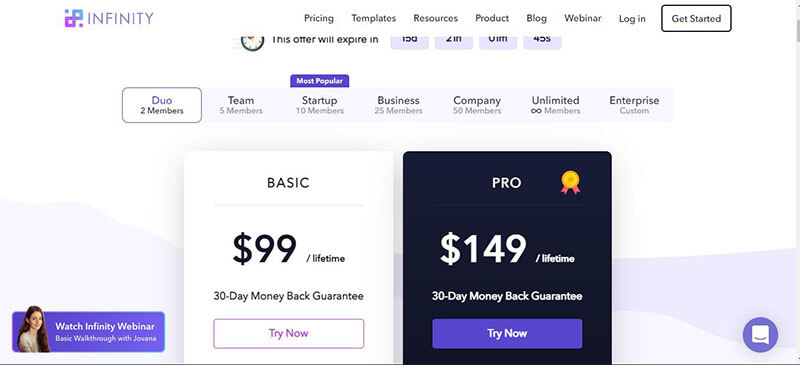The image depicts a screenshot of the Infinity website. In the top left-hand corner, the Infinity name and logo are prominently displayed. A navigation menu stretches across the top of the screen, including options such as Pricing, Templates, Resources, Product, Blog, Webinar, and Login. Notably, there is a "Get Started" button highlighted with a box to draw attention.

Several offers are presented prominently in the main section of the screen. One option is the Basic package, available for a lifetime fee of $99, which includes a 30-day money-back guarantee. Another option is the Pro version, priced at $149 for a lifetime, also with a 30-day money-back guarantee. The Pro version appears to be selected, as indicated by a call-to-action button labeled "Try Now."

In the left-hand corner, there is a link to watch an Infinity webinar, which offers a basic walkthrough of the platform. Directly above this, several membership options are detailed, ranging from two members, five members, 10 members, 25 members, 50 members, to an Infinity membership, with an option to specify a custom number of members.